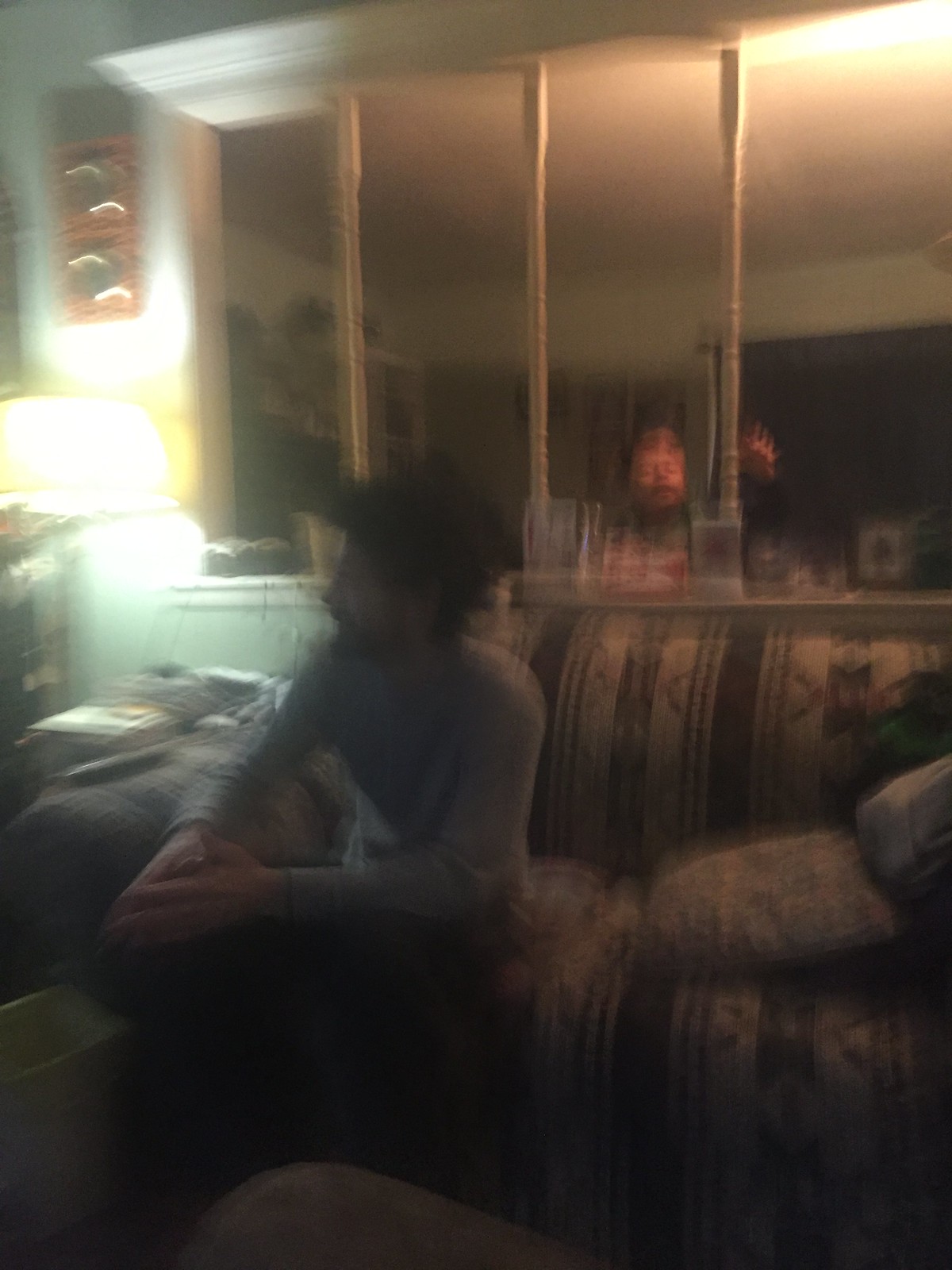The photograph, although very out-of-focus, depicts a man with a beard sitting on a small sofa adorned with brown and tan striped patterns interspersed with small geometric designs. He is dressed in a long blue shirt and appears to have his hands resting on his knee, folded together. Adjacent to his right leg is a small white waste bin. To his right, a bright light illuminates part of the scene. The man gazes towards this direction. In the background, another individual is visible, either looking straight ahead or downwards, engaged in an indeterminate activity. The room behind them is dimly lit, with a ceiling that has a pinkish-tan hue.